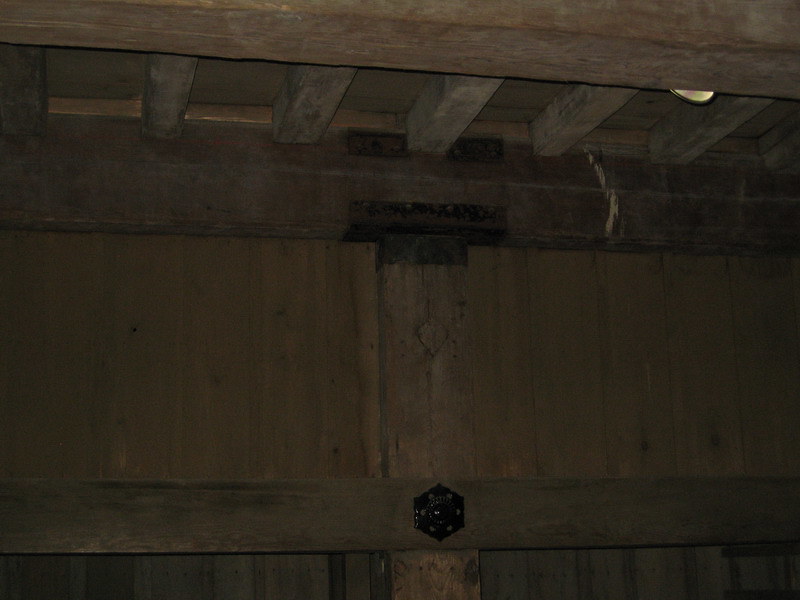This image depicts a dimly lit and aged wooden enclosure, potentially the interior of an old barn or similar structure. The scene features a dark brown wooden wall occupying the bottom three-fourths of the image, with visible rafters or support beams extending upwards to the ceiling in the top fourth. These beams run vertically and horizontally, forming a cross-pattern supporting the semi-visible wooden ceiling.

Prominently centered on one of the wall beams is an old, black metal piece, which could be a spigot, and resembles a hexagon with its six sides. This metal piece, along with several other black brackets scattered throughout the structure, is corroded and rusted, suggesting significant age—possibly 30 to 50 years or more. The wooden materials exhibit a range of light and dark brown hues, further emphasizing the structure's vintage and weathered appearance. The general setting evokes a sense of historical rustic charm, with its robust but time-worn wooden architecture.